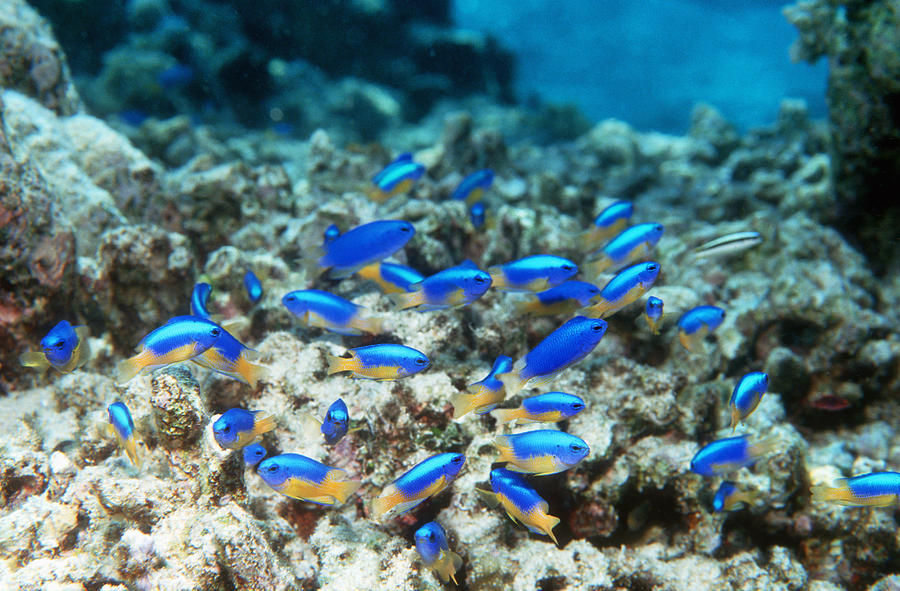This underwater photograph captures a vibrant school of approximately 20 small fish swimming in various directions. The fish are predominantly blue with bright yellow underbellies and tail fins, creating a striking contrast in the image. Their black eyes add fine detail to their lively appearance. In the foreground, the fish are sharply detailed, standing out against a backdrop that becomes progressively hazy. The underwater scape features a rocky or coral surface that ranges in color from white and tan to brown, fading into blues and greens and culminating in a deep blue towards the top. Coral formations are scattered across the ground, appearing slightly blurred, and giving depth to the scene. The upper portion of the image is tinged with a white-blue hue, indicative of the water's coloring. Notably, there is one fish on the right-hand side that is white with a dark stripe, adding a unique element to the composition.